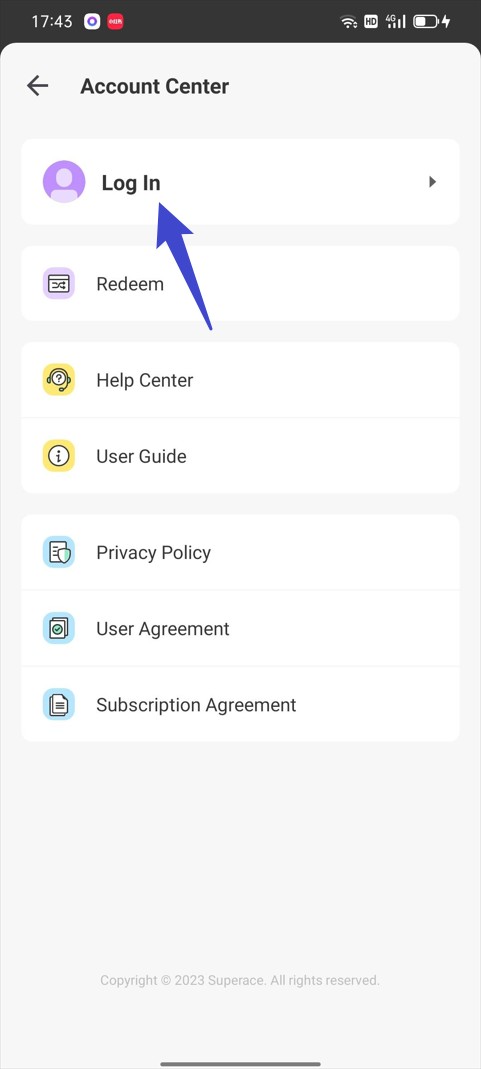The image depicts the "Account Center" section within the settings app on a Samsung phone. The background is a light gray, almost white in color, and the top of the screen includes a black status bar displaying crucial indicators like the time, battery icon, Wi-Fi icon, and mobile signal icon.

Nestled beneath this status bar is the title "Account Center," alongside a back arrow for navigation. The app's layout features a series of white rectangular sections, each containing specific text and icons aligned to the left. 

The top section labeled "Login" is distinguished by a purple arrow pointing towards it. Following this, the second section reads "Redeem" accompanied by an icon on a purple background.

Further down, in subsequent sections separated by some spacing, the items "Help Center" and "User Guide" are displayed, each associated with an icon on a yellow background. 

Toward the bottom, the sections "Privacy Policy," "User Agreement," and "Subscription Agreement" appear, each with an icon on a bluish background. 

The screen contains empty gray space below these sections, and at the very bottom, it states "Copyright 2023 Super Ace. All rights reserved."

![Samsung Account Center](#)